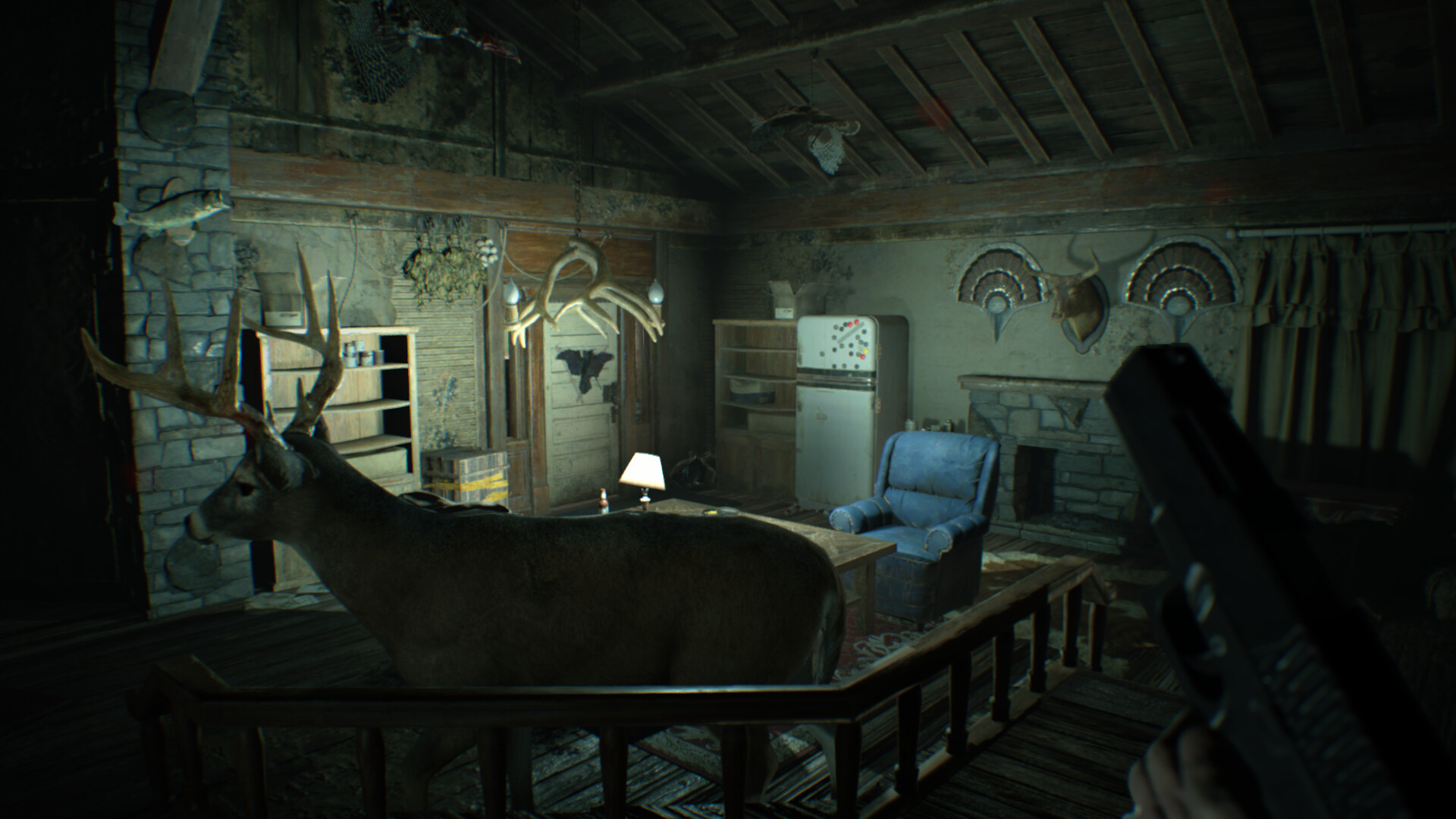The image appears to be a detailed scene from a role-playing game, capturing an immersive interior space. In the lower right corner, a partial view of a weapon and the character's left hand is visible, with fingers lightly gripping the handle. The character stands near a raised balcony or platform with dark brown wooden railings and visible spokes.

The scene features intricate decor including a realistic stuffed deer with prominent antlers, mounted on the wall near a stone-clad fireplace. The fireplace stones have a grid-like pattern, and above it, a mounted fish adds to the rustic ambiance. A pillar extends from the fireplace to the roof, supporting and connecting the structure.

In tandem with the fireplace, horizontal wooden beams support adjacent walls, forming a 90-degree angle with vertical purlins reaching up to another horizontal beam further up near the roof. A mounted bull's head is prominently displayed on one of the walls, contributing to the overall aesthetic.

Additional elements in the room include a white refrigerator, a tan-colored door, a bookshelf, and a blue recliner chair positioned near a wooden coffee table. A lamp with a white shade sits atop the coffee table, completing the cozy and meticulously detailed scene.